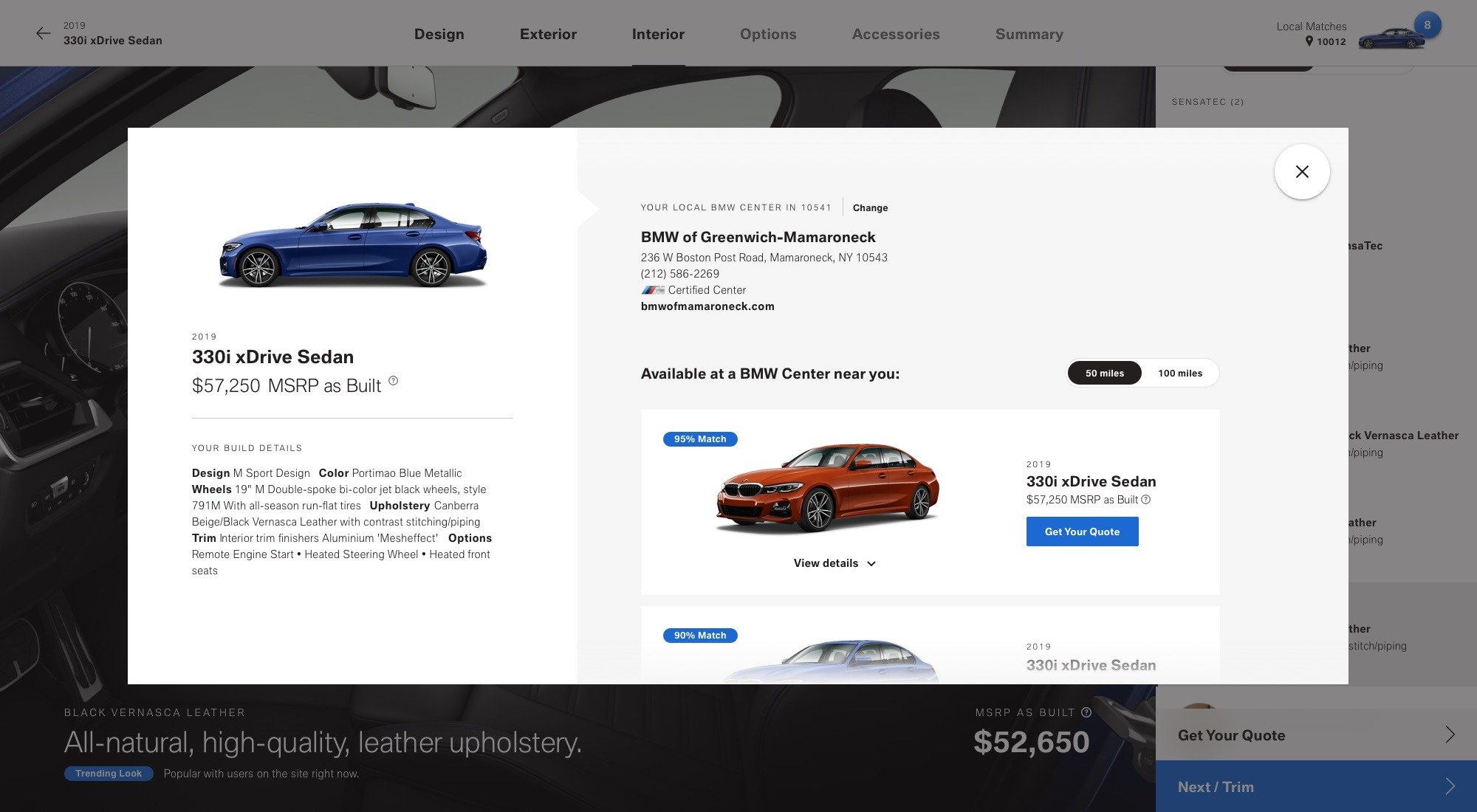### Detailed Caption:

This image captures a screenshot of a BMW webpage featuring the 2019 BMW 330i xDrive Sedan prominently at the top. Overlaid on the main page is a pop-up displaying the model details, including its name and MSRP of $57,250.

#### Main Content of the Page:
- **Vehicle Highlight:** 2019 BMW 330i xDrive Sedan.
- **Pricing Information:** MSRP as built: $57,250.
- **Build Specifications:** Main pop-up highlights build details regarding design, color, wheels, upholstery, options, and trim.
- **Local Dealership Information:** Below the vehicle details, there is information related to the local BMW Center, with the example provided being BMW of Greenwich located in Mamaroneck, NY, though the exact address and phone number are unreadable in the image.

#### Page Navigation and Other Elements:
- **Interior Photograph:** The background features an image showcasing the luxurious interior of the vehicle.
- **Tabs on the Main Page:** Behind the pop-up overlay, the webpage contains interactive tabs labeled "Design," "Exterior," "Interior," "Options," "Accessories," and "Summary" for easy navigation through the car's features.
- **Distance Options:** There are dropdowns to select dealership options within different mile ranges, specifically 50 miles and 100 miles.
- **Additional Visuals:** Another smaller photograph of the BMW 330i xDrive Sedan can be seen, with a dropdown arrow indicating that more details can be accessed by interacting with it.

Overall, the webpage is a comprehensive overview of the 2019 BMW 330i xDrive Sedan, providing both build customization options and local dealership information for potential buyers.